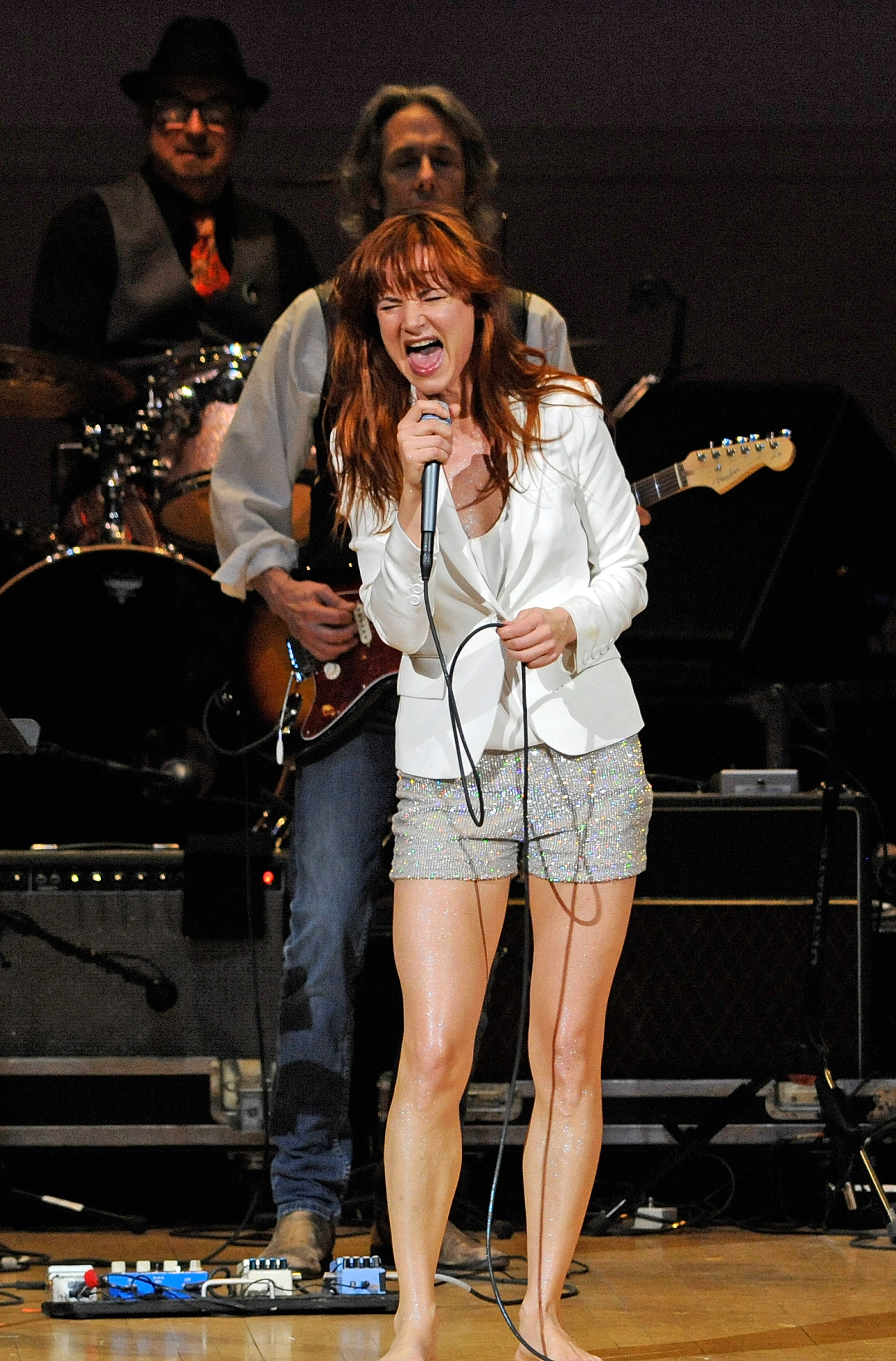This vibrant color photograph captures an energetic live performance scene. Dominating the foreground is a dynamic female singer, who might be actress Juliette Lewis or simply bears a striking resemblance to her. She is fervently singing into a gray metallic microphone, grasped in her right hand, with its long wire trailing down. Her lustrous, long reddish-brown hair flows wildly as she belts out the music.

She is attired in gray shorts that expose her bare legs, and she stands barefoot on the beige-tiled stage, exuding a raw and authentic rock vibe. 

Behind her, a variety of guitar pedals lie on the floor, integral to the electric guitar setup. To her rear, a guitarist clad in a white shirt and a vest is fervently playing an electric guitar, adding layers of sound to the performance.

Further back, the drummer, dressed in a gray vest over a black shirt, accented by a red tie, black hat, and glasses, is passionately playing a drum set, contributing to the powerful rhythm driving the act. The collective focus and intensity of the musicians create an electrifying ambiance, encapsulating the essence of live rock performance.